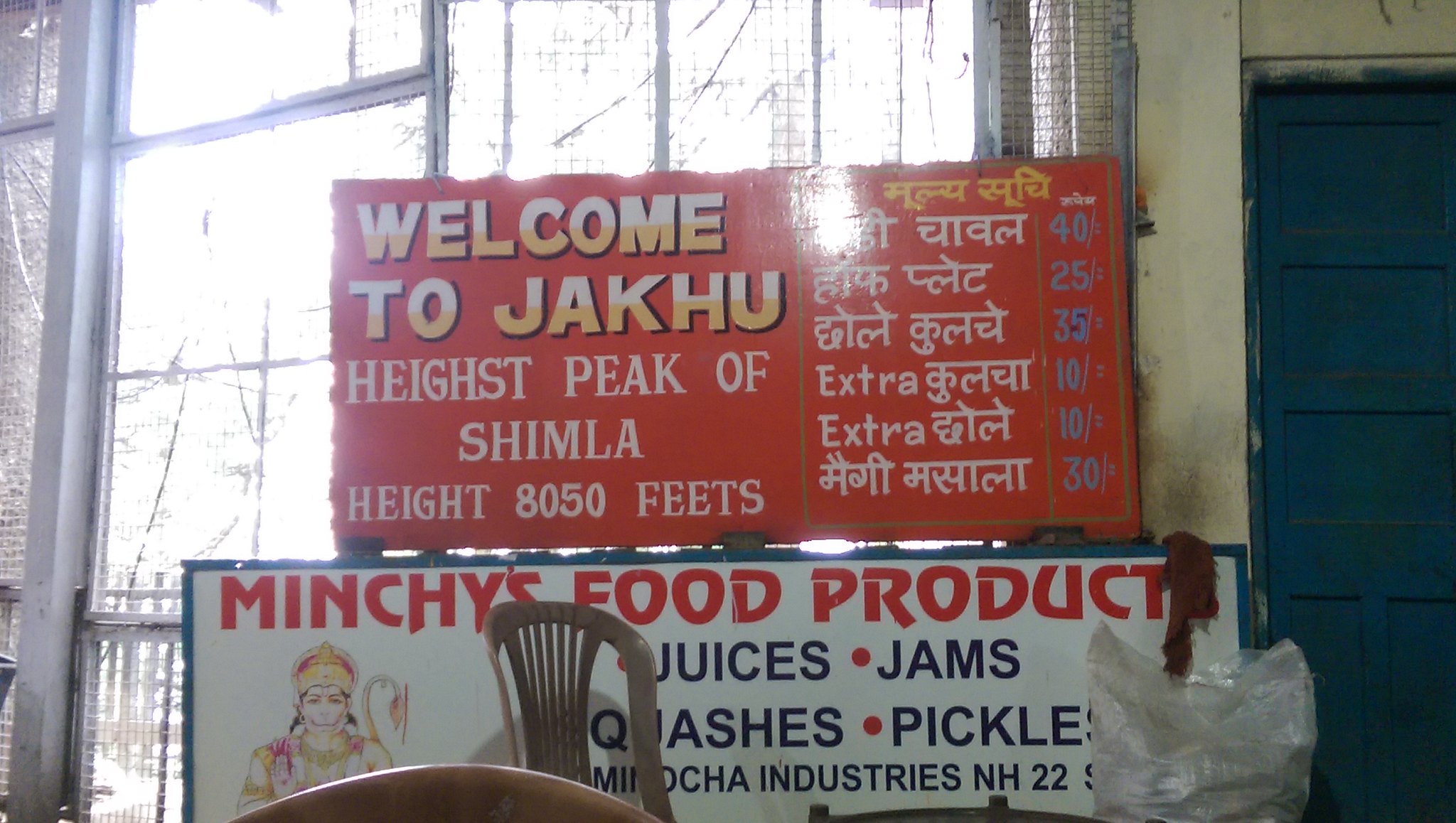This indoor photograph captures a quaint, somewhat dilapidated setting characterized by a mix of brick and white walls, with a prominent blue door on the right that has noticeably poorly painted trim. Centered in the image is a detailed sign with a gray background that reads "Welcome to Jakku, highest peak of Shimla, height 8,050 feet." This text is accompanied by what appears to be additional information in either Chinese or Japanese, followed by a series of numbers: 40, 25, 35, 10, 10, 30. Below this, another sign advertises "Minchi's Food Products" offering various items such as juices, jams, squashes, and pickles, from Minocha Industries NH22, and features a character on the left side of the sign. The background includes a large window, through which branches of trees and sunlight can be seen, adding to the slightly run-down but cozy ambiance. The mention of "metal wiring" on the window and the potential impression of cracks, possibly caused by thin tree branches outside, further accentuates the rustic feel of the space.